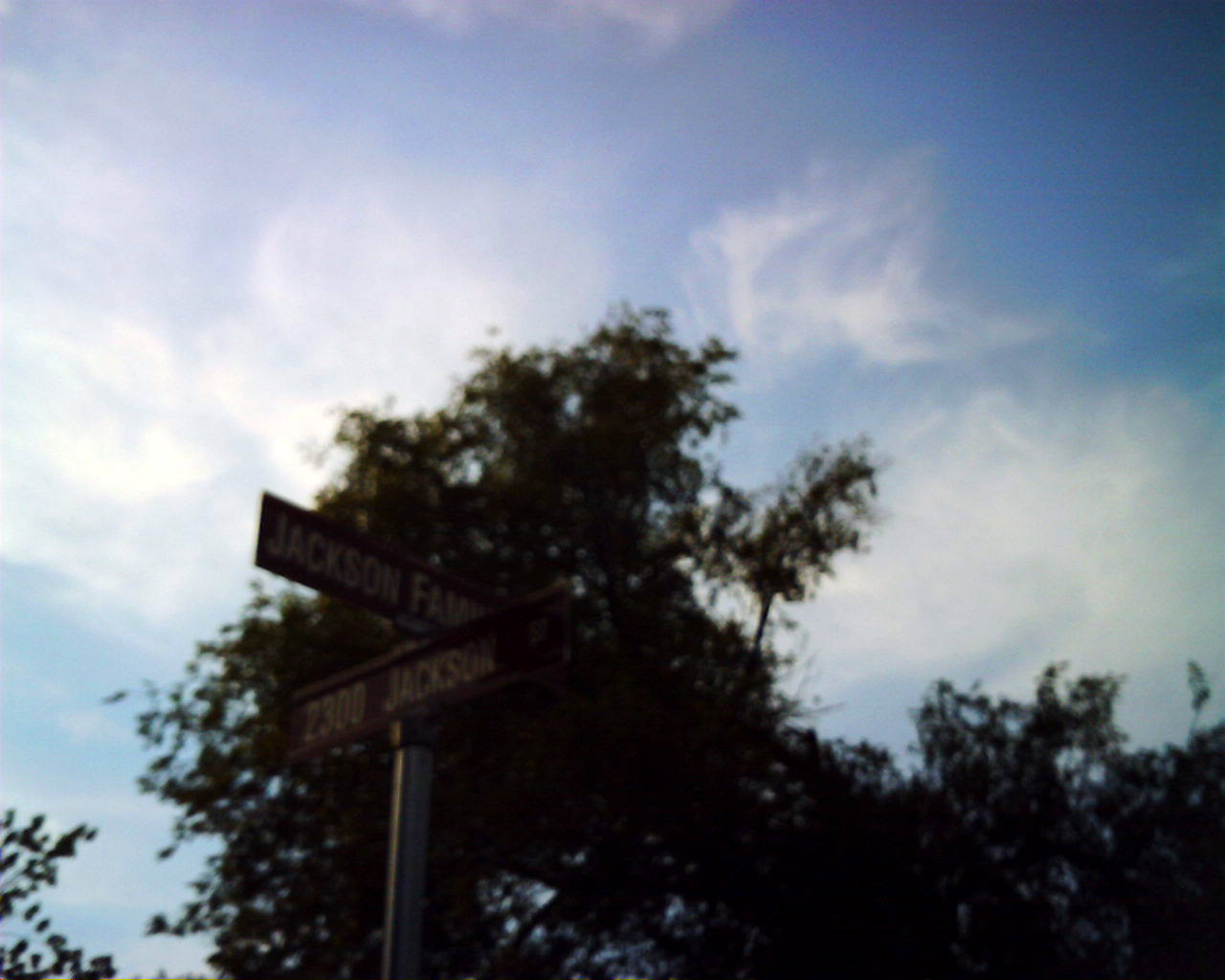This photograph captures a street sign intersection from an upward angle, framed against a backdrop of lush treetops. At the top of the metal pole, a brown, rectangular sign with white text reads "Jackson Fam" with the final letters partially cut off, possibly intended to say "Jackson Family." Directly below, another brown street sign, also with white text, indicates "2300 Jackson." The natural scenery of tree canopies provides a serene background contrast to the urban street signs.